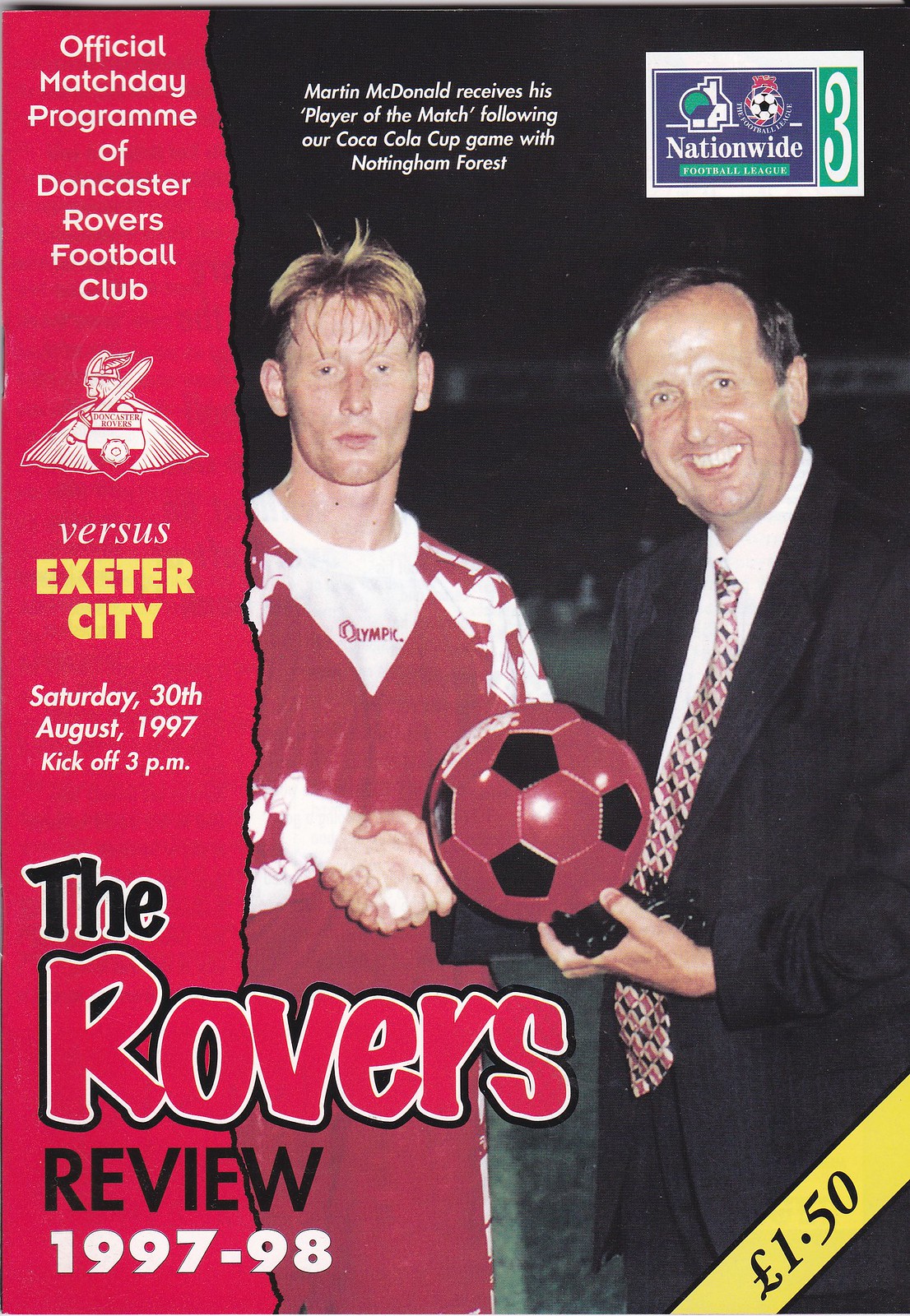This image depicts the cover of "The Rovers Review," the official match day program of Doncaster Rovers Football Club. The left side features a vertically torn red banner with white text, stating "Official match day program of Doncaster Rovers Football Club." Below this, the club's Viking logo, adorned with a helmet and sword, is displayed alongside a red and white badge followed by the text "Versus Exeter City, Saturday 30th August 1997, kickoff 3 p.m." At the bottom, large text reads "The Rovers Review 1997 to 98," with "Rovers" in red outlined in black.

On the right side, a photograph captures a footballer with short blonde hair, wearing a red and white jersey, shaking hands with a smiling man in a black suit, white shirt, and checkered tie who is holding a red and black football. The footballer's expression is notably distant. Above this image, in white text, it states, "Martin McDonald receives his player of the match following a Coca-Cola cup game with Nottingham Forest." The top right corner displays a logo of the Nationwide Football League 3. In the bottom right corner, a yellow diagonal banner with black text marks the price as "One pound fifty."